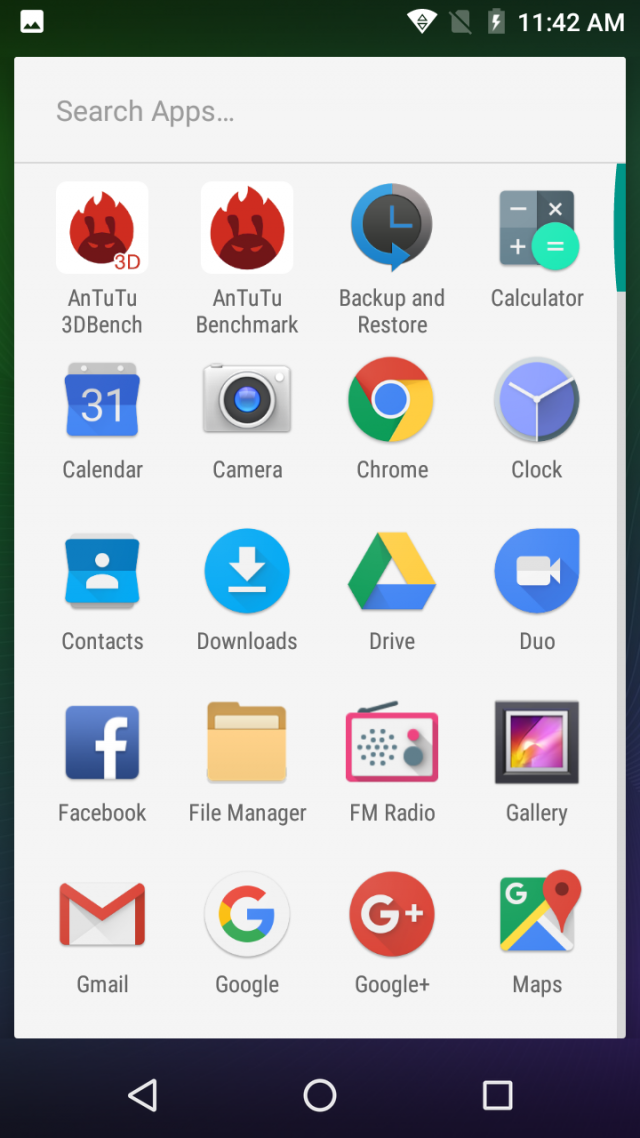The image displays a screenshot of an Android smartphone. At the top of the screen, the status bar contains various icons: a square icon with rounded corners showing two mountain peaks of different heights, the Wi-Fi symbol with up and down arrows inside it, and a rectangle with a backslash through it. Additionally, there's a battery icon with a lightning bolt, indicating the battery is charging, and the current time displayed as 11:42 a.m.

Directly below the status bar is a text box labeled "Search apps," indicating that the user is on a screen dedicated to searching for apps. Following this, the screen shows 20 app icons organized in a grid consisting of four columns and five rows. Specific app icons visible include Antutu 3D Bench, Antutu Benchmark, Backup and Restore, Calculator, Calendar, Camera, Chrome, Clock, Contacts, Downloads, Drive, Duo, Facebook, File Manager, FM Radio, Gallery, Gmail, Google, Google+, and Maps.

At the bottom of the screen, the navigation bar is visible, showing the standard Android navigation icons: a triangle for back, a circle for home, and a square for recent apps.